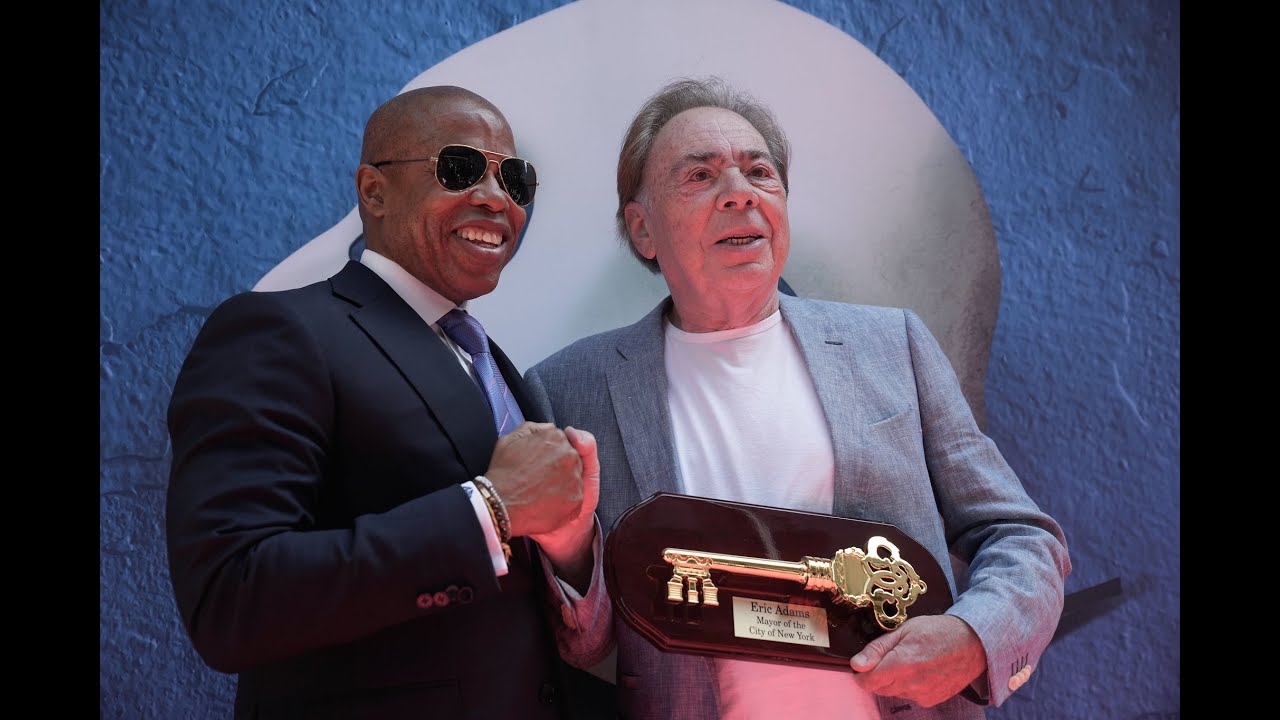In this celebratory image, two men are prominently featured, shaking hands and smiling. On the left is Eric Adams, the African-American Mayor of New York City, who is distinguished by his dark suit, white shirt, blue tie, and aviator sunglasses. He is happily presenting a ceremonial key to the city. On the right stands an older white gentleman with gray hair, dressed in a light gray suit jacket over a white t-shirt. He appears to be in his 70s and is holding a plaque featuring a large golden key, inscribed with Mayor Adams' name. The backdrop consists of a blue textured wall with a noticeable white circular object partially obscured by the men. The edges of the image have black strips, framing the communal display of honor and celebration.